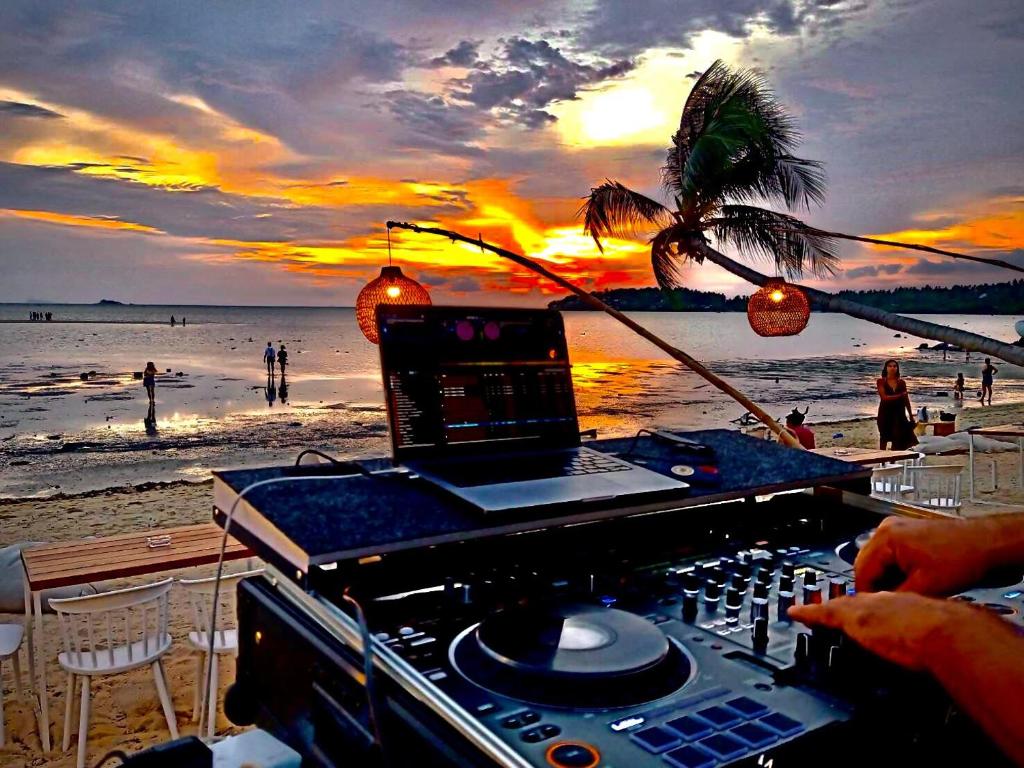The photograph captures a vibrant and energetic outdoor scene featuring a DJ setup on a beach at sunset. Dominating the bottom half of the image is a black, boxy DJ mix table, dotted with various black knobs and buttons, which is being adjusted by the DJ's hands. On a slightly raised platform on the same device rests a white and black laptop, from which white wires extend to connect with the rest of the equipment. 

In the background, the tan-colored sandy beach is kissed by blue ocean waves, creating a serene yet dynamic backdrop. The sky above is a stunning gradient of orange hues, indicating a setting sun. 

Adding to the lively atmosphere, there are several white chairs and brown tables scattered around, with people occasionally visible in the scene. Off to the side, a bent palm tree and additional chairs and tables further enhance the tropical setting. Two lights hung on tall poles suggest that the area might be prepared for continued festivities into the evening. 

The major colors in the image include black, white, tan, blue, orange, yellow, brown, and shades of green, forming a rich and inviting visual palette without any visible text.